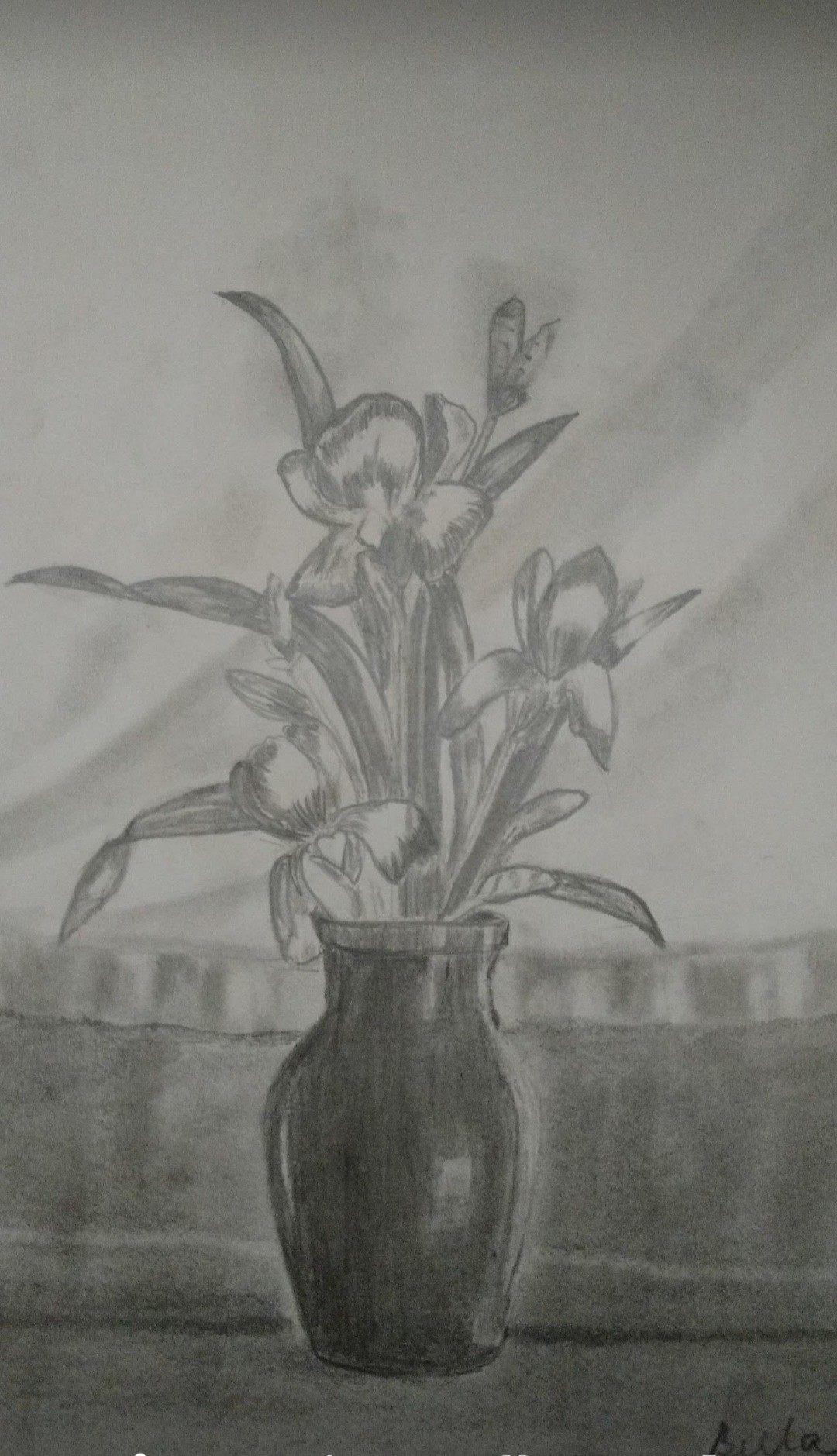This black and white drawing features a detailed depiction of a flower vase filled with various flowers and plants. The vase, located centrally and towards the bottom of the composition, is rendered in black. The intricate line work showcases the delicate and diverse nature of the flowers and foliage contained within the vase. In the bottom right corner, a blurry black initial can be faintly observed, though it is difficult to discern clearly due to its indistinctness. The background transitions from a dark, black hue at the bottom to a lighter, white shade with subtle black accents above, adding depth and contrast to the artwork. Overall, the composition is focused solely on the vase and its contents, with no other elements present in the scene.